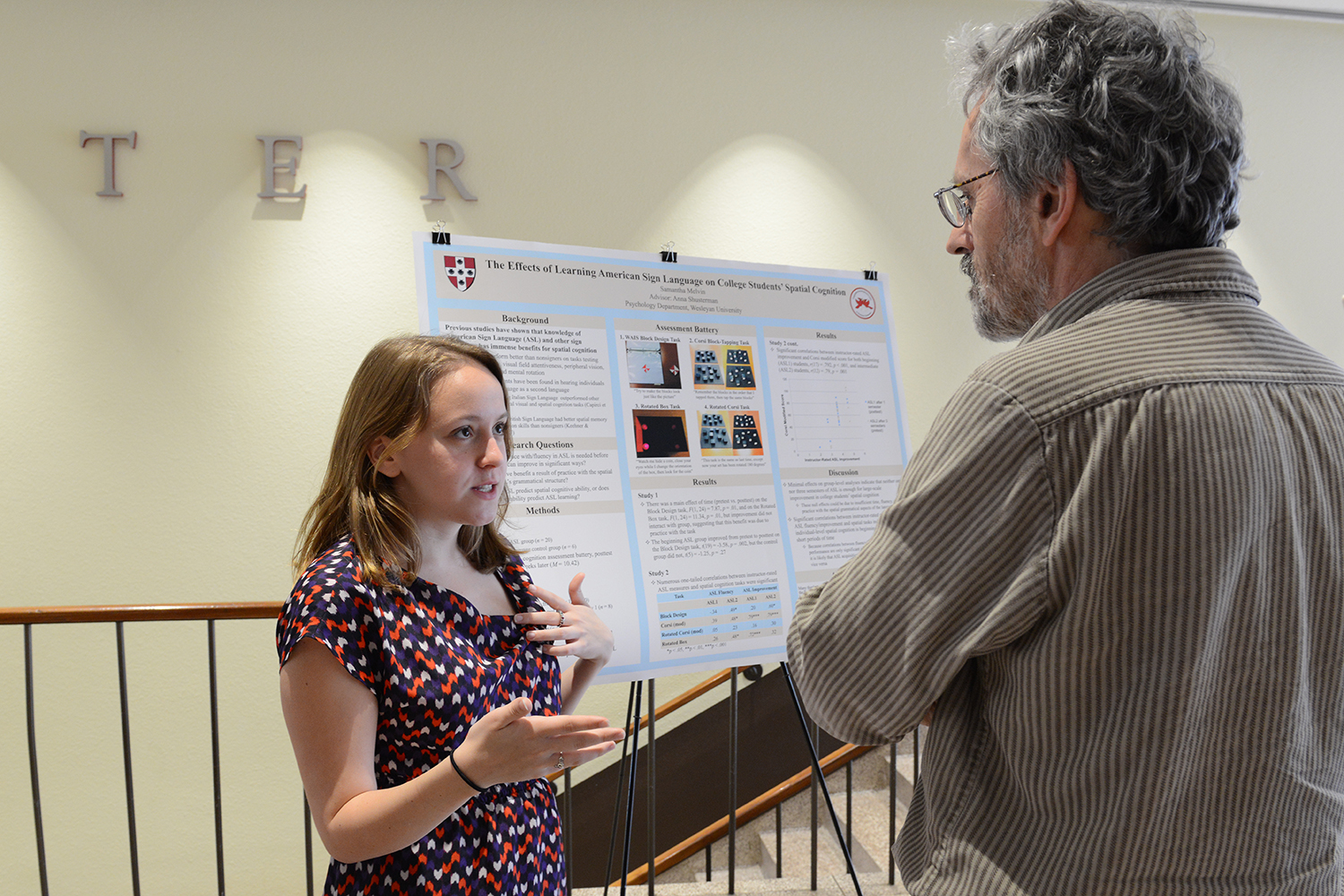In this vibrant photo taken at what appears to be a science fair or similar academic event, a young female student dressed in business casual attire engages in an animated discussion with an elderly gentleman, likely her professor or a mentor. The girl, who seems to be around 12 or 13 years old, is captured mid-presentation with her hands in expressive motion and a serious expression on her face. Behind her, a meticulously crafted poster board sits on an easel, detailing her research on "The Effects of Learning American Sign Language on College Students' Spatial Cognition." The professor, an older man with gray hair and glasses, listens attentively, dressed in a striped, collared shirt and khakis. The presentation setup is situated near a staircase, adding to the academic ambiance of the setting. The detailed poster board, although somewhat blurry, showcases sections on questions, methods, results, and assessment battery, underscoring the depth and significance of her work in this specialized topic.